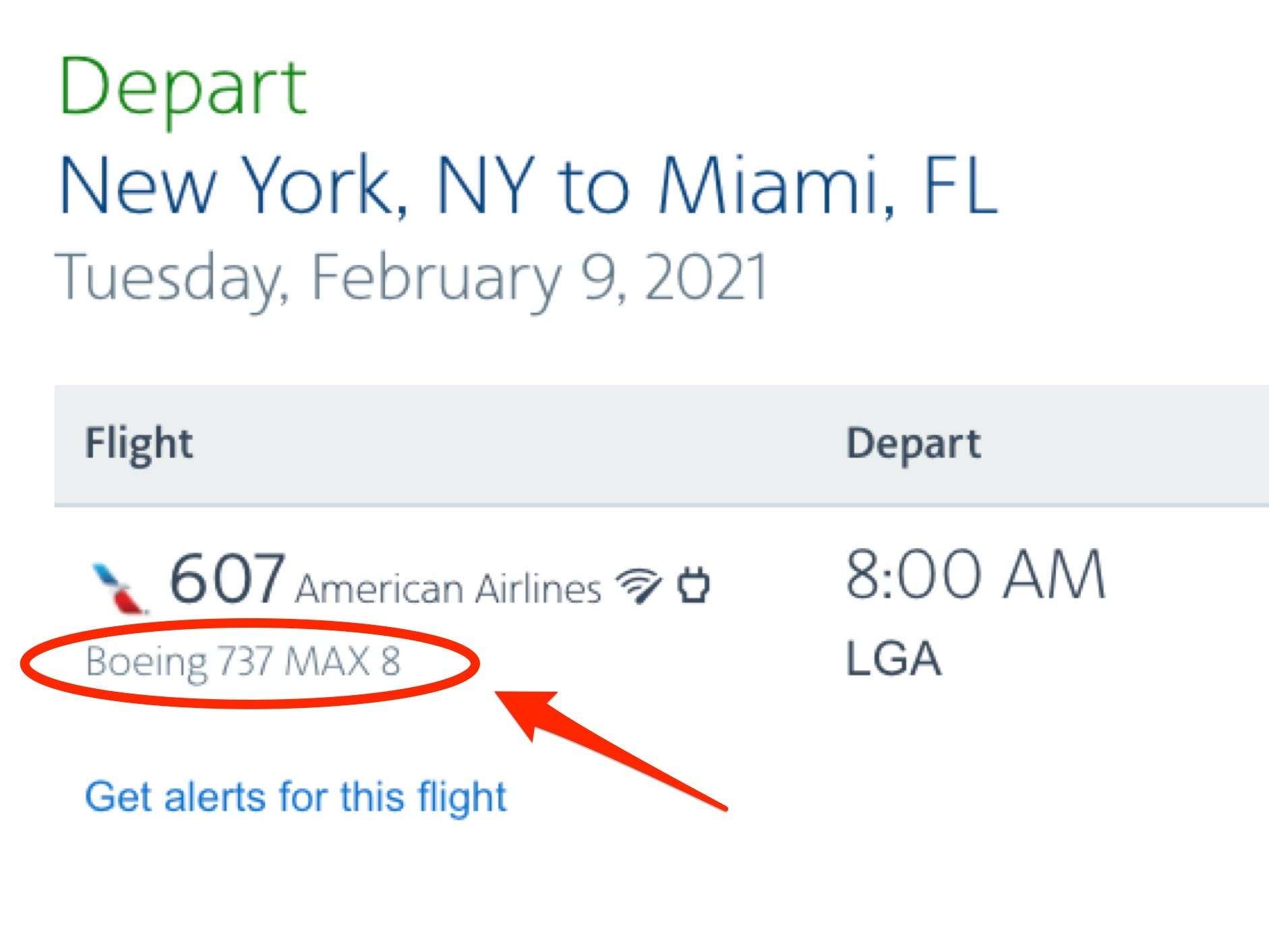Screenshot of a webpage displaying flight details for a departure from New York to Miami on Tuesday, February 9th, 2021. The highlighted flight, American Airlines Flight 607, departs from LaGuardia Airport (LGA) at 8:00 a.m. The flight will be operated by a Boeing 737 MAX 8, which is circled in red and accompanied by a red arrow pointing to it. Notably, the Boeing 737 MAX 8 model is highlighted due to its controversial history involving safety issues and ongoing legal matters concerning Boeing. Additional details on the page include an option to set up flight alerts in blue text, and indications that Wi-Fi and power charging are available on board. The page primarily serves to inform passengers about the specific departure time and aircraft model for this particular flight.